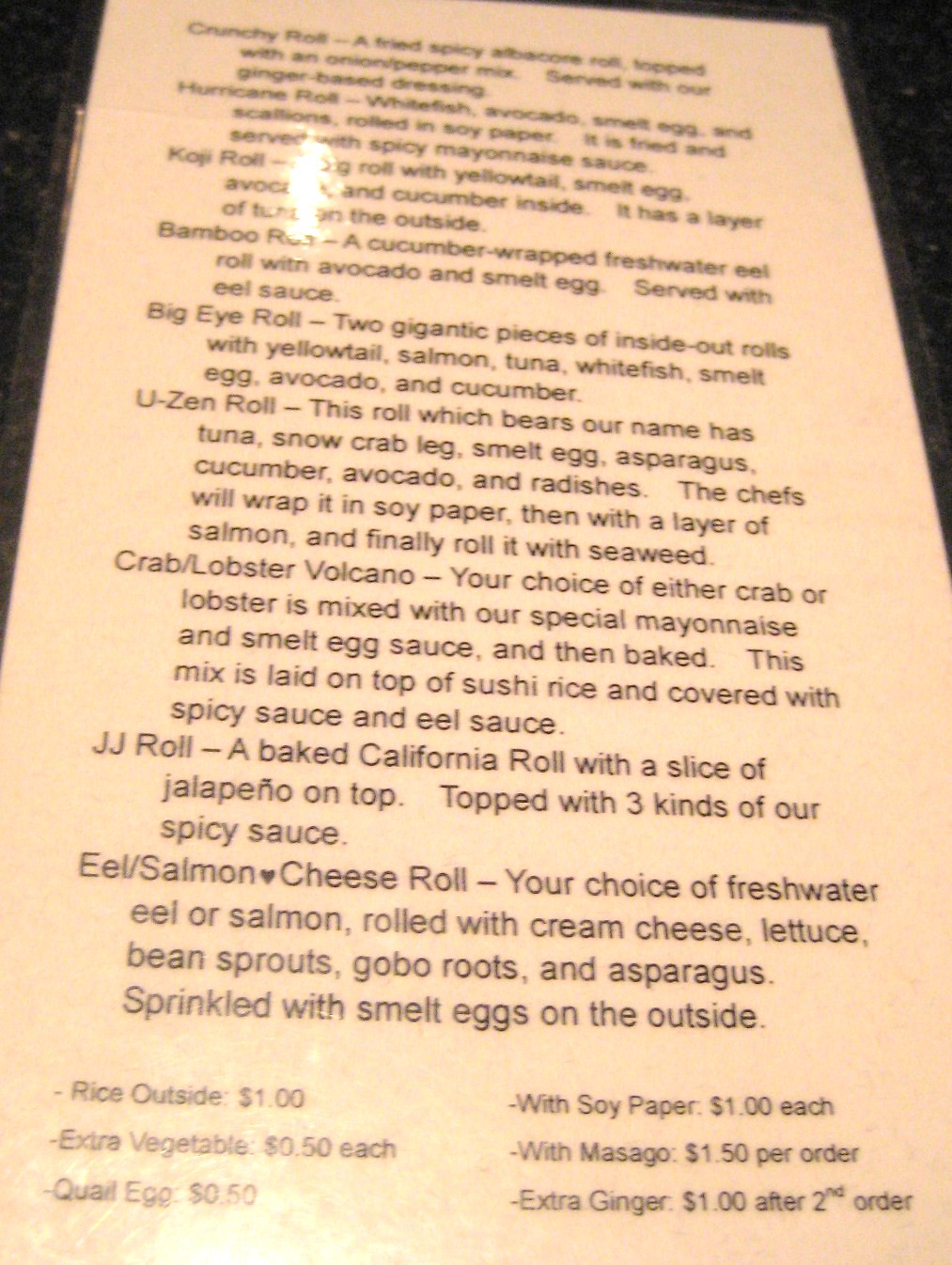In this photograph, a large, detailed menu is prominently displayed, featuring a variety of food items. At the top of the menu is the "Crunchy Roll," described as a fried spicy artichoke roll topped with onions and a pepper mix, served with a unique gingerbread dressing. Next is the "Hurricane Roll," consisting of white fish, avocado, smelt egg, and scallions rolled in soy paper, fried, and served with spicy mayonnaise sauce.

The "Koji Roll" follows, which includes yellowtail, smelt egg, avocado, and cucumber inside, with an exterior layer of tuna. The "Bamboo Roll" is a cucumber-wrapped freshwater eel roll with avocado and smelt egg, served with eel sauce. The "Big Eye Roll" is highlighted as two substantial inside-out rolls filled with yellowtail, salmon, tuna, white fish, smelt egg, avocado, and cucumber.

The "Cousin Roll," which carries the restaurant’s namesake, includes tuna, snow crab legs, smelt egg, asparagus, cucumber, avocado, and radishes, all wrapped in soy paper, layered with salmon, and finally encased in seaweed. 

Towards the end of the menu, items such as the "Crab Lobster Volcano," "JJ Roll," and "Eel Salmon Cheese Roll" are listed. The "Eel Salmon Cheese Roll" offers a choice between freshwater eel or salmon combined with cream cheese, lettuce, bean sprouts, gabo roots, and asparagus, with smelt eggs sprinkled on the outside.

The bottom of the menu includes additional options and pricing: rice on the outside for $1, extra vegetables for $0.50, quail egg for $0.50, soy paper for $1, masago for $1.50 per order, and extra ginger for $1 after the second order.